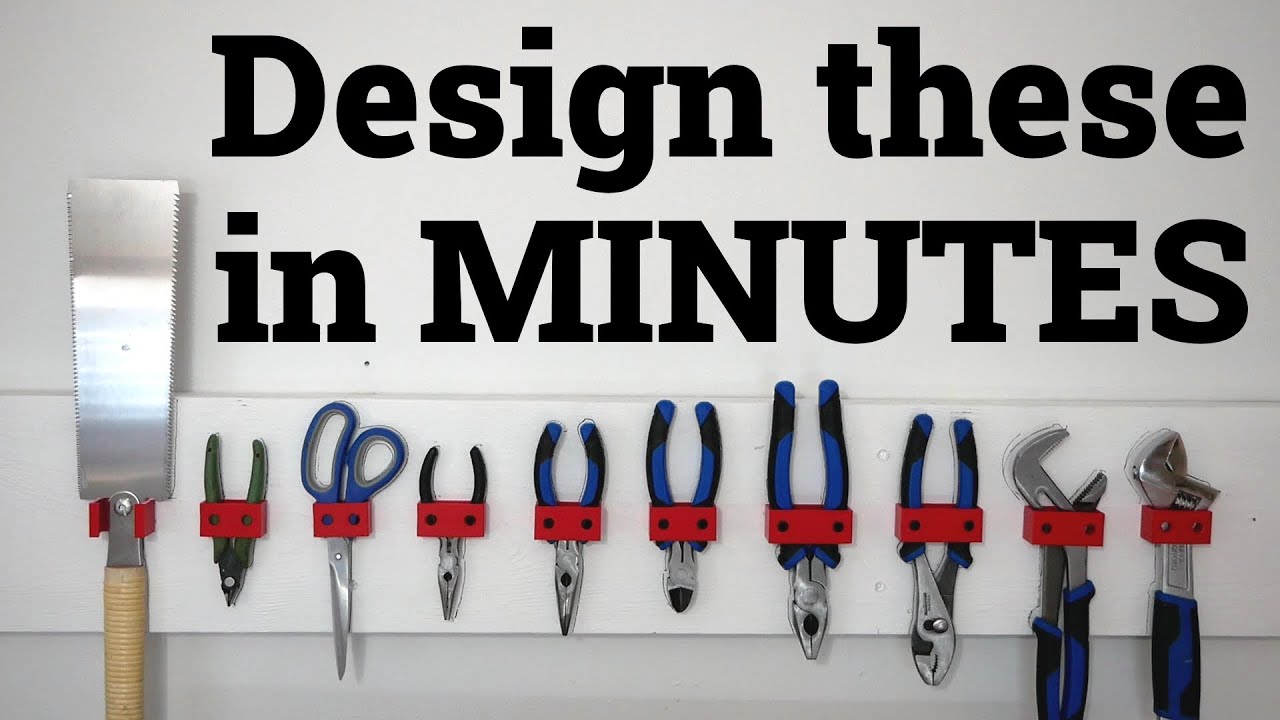The photograph captures a detailed and organized display of various tools hanging from fixtures on a white-painted wooden plank that's screwed into a white wall. At the top of the image, bold black text commands attention with the phrase "DESIGN THESE IN MINUTES," emphasizing the word "MINUTES" in all capitals. The tools are neatly arranged and include a selection of pliers, a pair of scissors, wire cutters, and plumbing wrenches, all featuring either blue or green handles. Specifically, from left to right, the tools include a long, flat hand saw with a serrated edge on both sides, wire snippers, a pair of scissors, needle nose pliers (both short and long), regular pliers with cutting edges, a pair of diagonal cutters, channel locks, and a crescent wrench. This setup provides a highly accessible and visually appealing way to organize tools for projects, making them readily available at a glance.